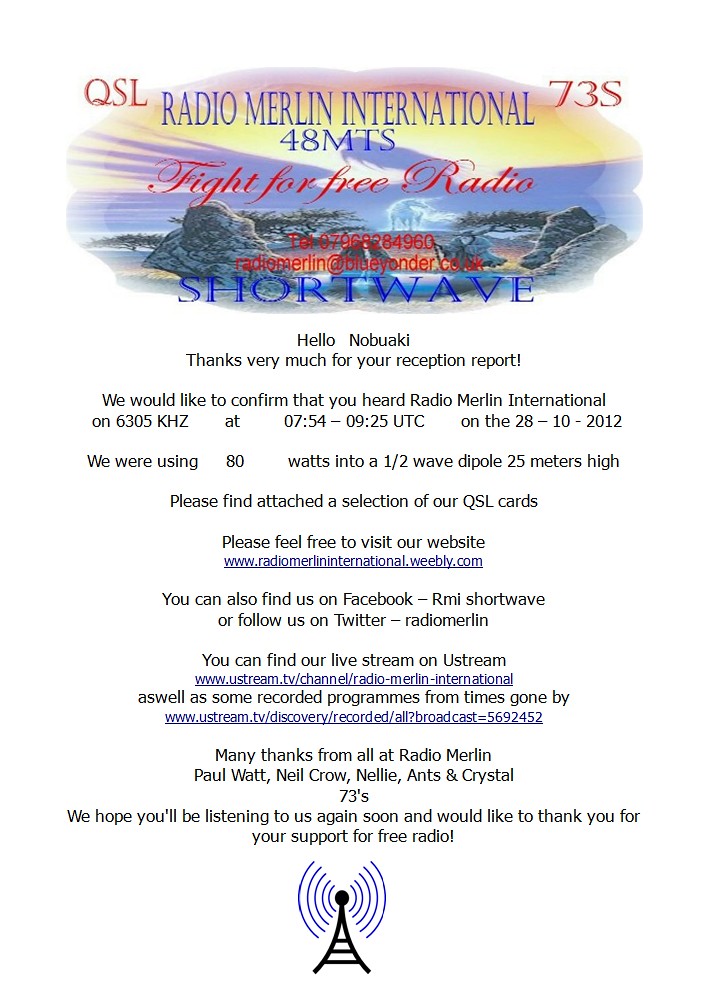The image is a poster with a white background featuring a winter fantasy landscape at the top, showing a sunset with purple and yellow skies, and a white unicorn among trees and rocks. The text near the top in blue reads "QSL Radio Merlin International, 48 MTS, fight for free radio, short wave." Below that, in a mix of black and blue text, it says, "Hello Nabuaki, thanks very much for your reception report. We'd like to confirm that you heard Radio Merlin International on 6305 kilohertz at 754 to 925 UTC on the 28th of October, 2012, using 80 watts into a half-wave dipole at 25 meters high. Please find attached a selection of our QSL cards. Many thanks from all at Radio Merlin." Additionally, there's some information about their live stream, website, and Facebook page along with a small logo of a radio tower at the bottom.